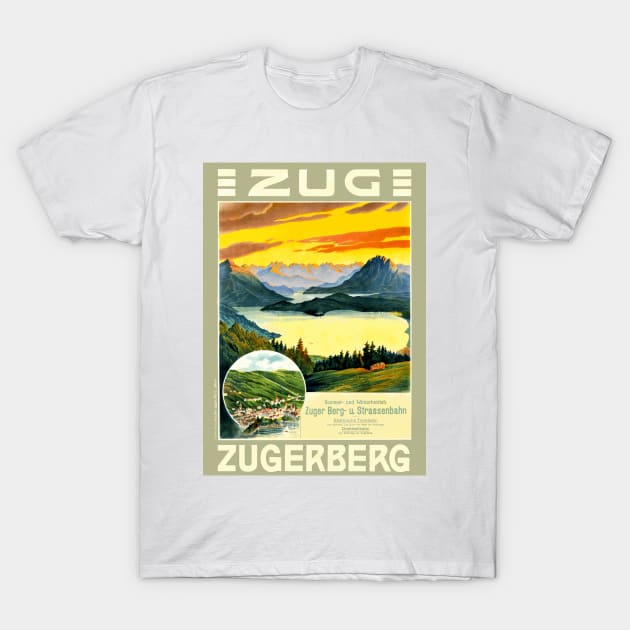This photograph showcases a plain white short-sleeved t-shirt laid flat on a white surface. The shirt features a large, vertical rectangular print on the chest area. The rectangle has a tan or greenish beige background, with three cream-colored, vertical dashes at the top. Just below the dashes, in prominent cream-colored letters, it says "ZUG, Z-U-G." The central part of the rectangle is dominated by a stylized painting of an alpine meadow leading to a serene lake, with majestic mountains in the background under an orange and yellow sunset sky. This artwork evokes the style of a 1950s travel poster with its vibrant greens, blues, and warm hues. At the bottom of the rectangle, in matching cream-colored text, it reads "ZUGERBERG, Z-U-G-E-R-B-E-R-G." There's also a small circle at the bottom of the artwork displaying a zoomed-in view of the actual area, which offers a detailed snapshot of a mountain scene. To the right of this circle, there is a small ivory or yellowish box with blue writing, adding additional details, possibly in German, describing the location or significance of the image.